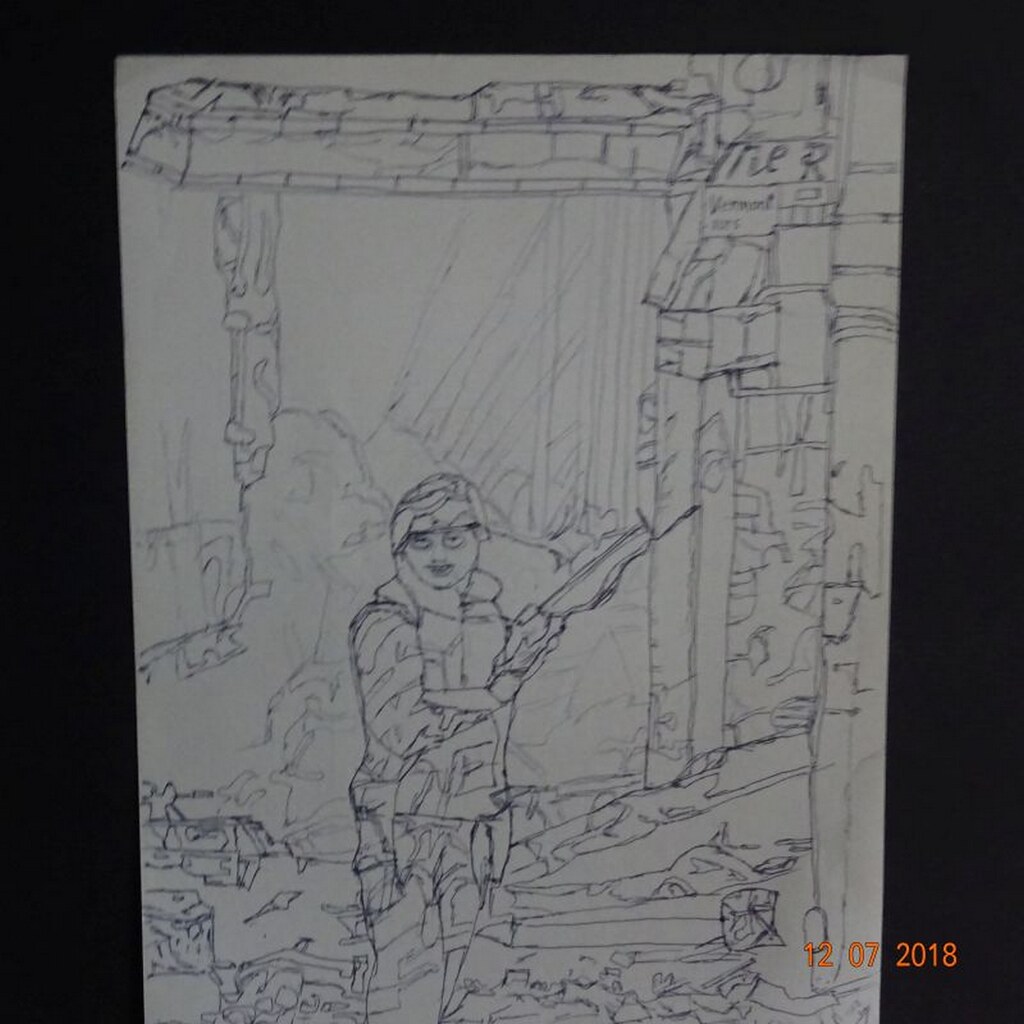The image is a digitized photograph of a hand-drawn picture, created with either pen or pencil on white paper. It depicts a soldier, likely female, without a helmet, holding a rifle in her right hand with a direct gaze, possibly showing a slight smile. The soldier appears to be wearing glasses and has long hair. Behind her is a structure made of blocks or bricks, resembling an entrance with a long, rectangular white feature on top. Scattered around is debris, suggesting a war zone setting. The background includes various shapes and sizes, some resembling buildings or columns. Additional details include faint text that spells "M-E-R" and a date stamp at the bottom right corner reading "12-07-2018". The image has black borders, indicating it was framed or formatted, likely captured by a digital camera.